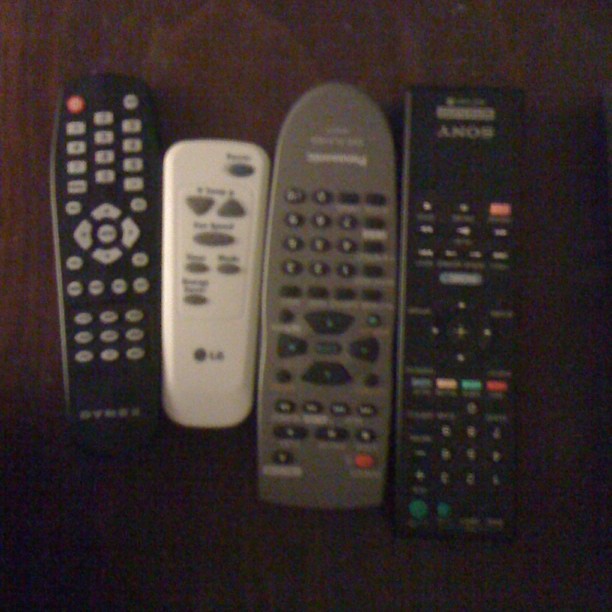In this fuzzy, low-lit color photograph, four distinct remote controls are laid out on a dark brown wooden table. From left to right, the first remote is black with gray buttons, bearing the faint and unreadable logo, potentially Sony. Next to it is a small white LG remote, most likely for a ceiling fan, with gray buttons. The third remote is light gray with black buttons and prominently features the Panasonic logo. On the far right is another black remote, distinctly marked with the Sony brand, characterized by white numbers and a few multicolored buttons. The remotes vary in shape and size, but the image quality makes it challenging to discern finer details.